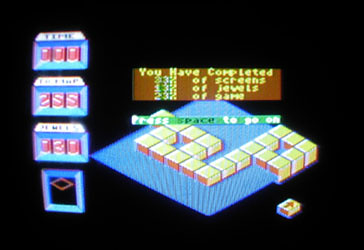The image displays a screenshot of an old-school, pixelated video game against a black background. Dominating the right side of the screen is a blue diamond-shaped board dotted with yellow blocks arranged in various patterns, including an eight-block square on the upper right that has a missing center. Additional blocks form snake-like patterns extending through the diamond. Above this graphic, there's a green rectangular panel with yellow text reading "Press SPACE to go on," and a brown rectangular bar at the top with a yellow message stating, "You have completed." This is followed by illegible numbers next to "of screens," "of jewels," and "of game," indicating player progress percentages. On the left side of the image, there are four vertically stacked rectangles, the top one labeled "Time," ostensibly showing game progress with fruit machine-like indicators. Red squares embedded in blue triangles, a blue square with a black and red diamond, further add to the complexity of the game's layout.